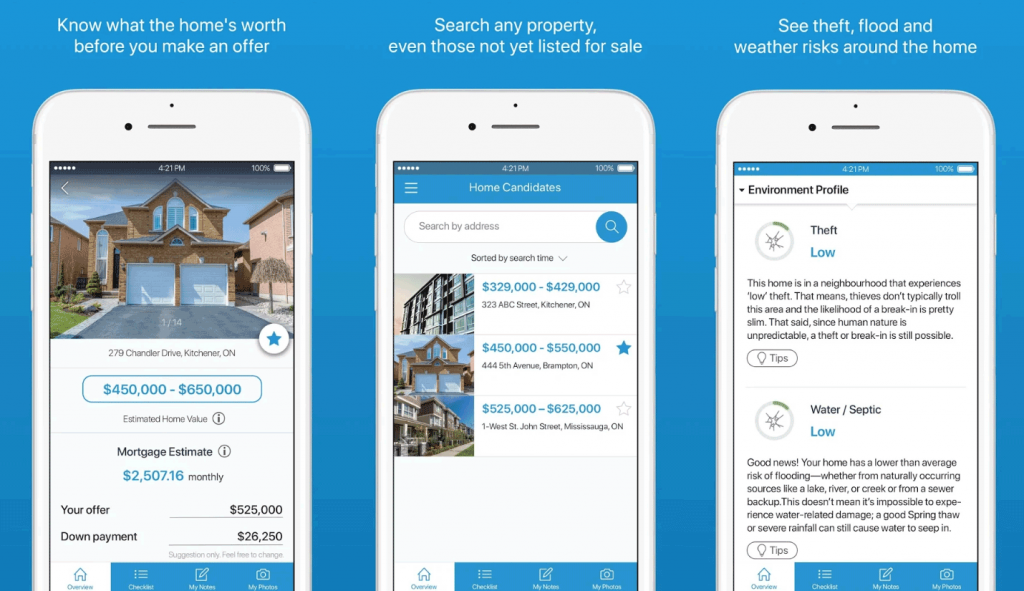The webpage features a blue background and is dedicated to helping users get the best deals on homes. In the top left corner, there's a headline stating, "Know what the home is worth before you make an offer."

Beneath the headline, there's an image of a cell phone displaying a photo of a brown two-story house with a two-car garage at the front. Below the house image, the text reads: "279 Chandler Drive, Kitchener, Ontario," followed by "Estimated Home Value: $450,000 to $650,000." Additional details provided include "Mortgage Estimate: $2,507.16 monthly," "Your Offer: $525,000," and "Down Payment: $26,250."

To the right of this text, there's another line that says, "Search any property, even those not yet listed for sale." This section contains another image of a cell phone screen. At the top of this screen, it reads "Home Candidates," accompanied by a search box with the text "Search by address" and a magnifying glass icon on the right. Below the search box, properties are listed as "Sorted by search time." The first listing features an image of a building exterior and states, "Estimated Value: $329,000 to $429,000," and "323 ABC Street, Kitchener, Ontario."

A smaller image shows the same house from the earlier display with new details: "Estimated Value: $450,000 to $550,000," and "444 Fifth Avenue, Brampton, Ontario." Another picture shows a few homes on a street along with the text, "Estimated Value: $525,000 to $625,000."

On the far right is a different cell phone screen showcasing environmental data for potential home buyers. Above it, the text reads, "See theft, flood, and weather risks around the home." On the screen, a section titled "Environmental Profile" highlights categories like "Theft" and "Water/Septic."

This comprehensive setup provides users with essential information to make well-informed decisions when purchasing a home, ensuring clarity and transparency in the real estate process.